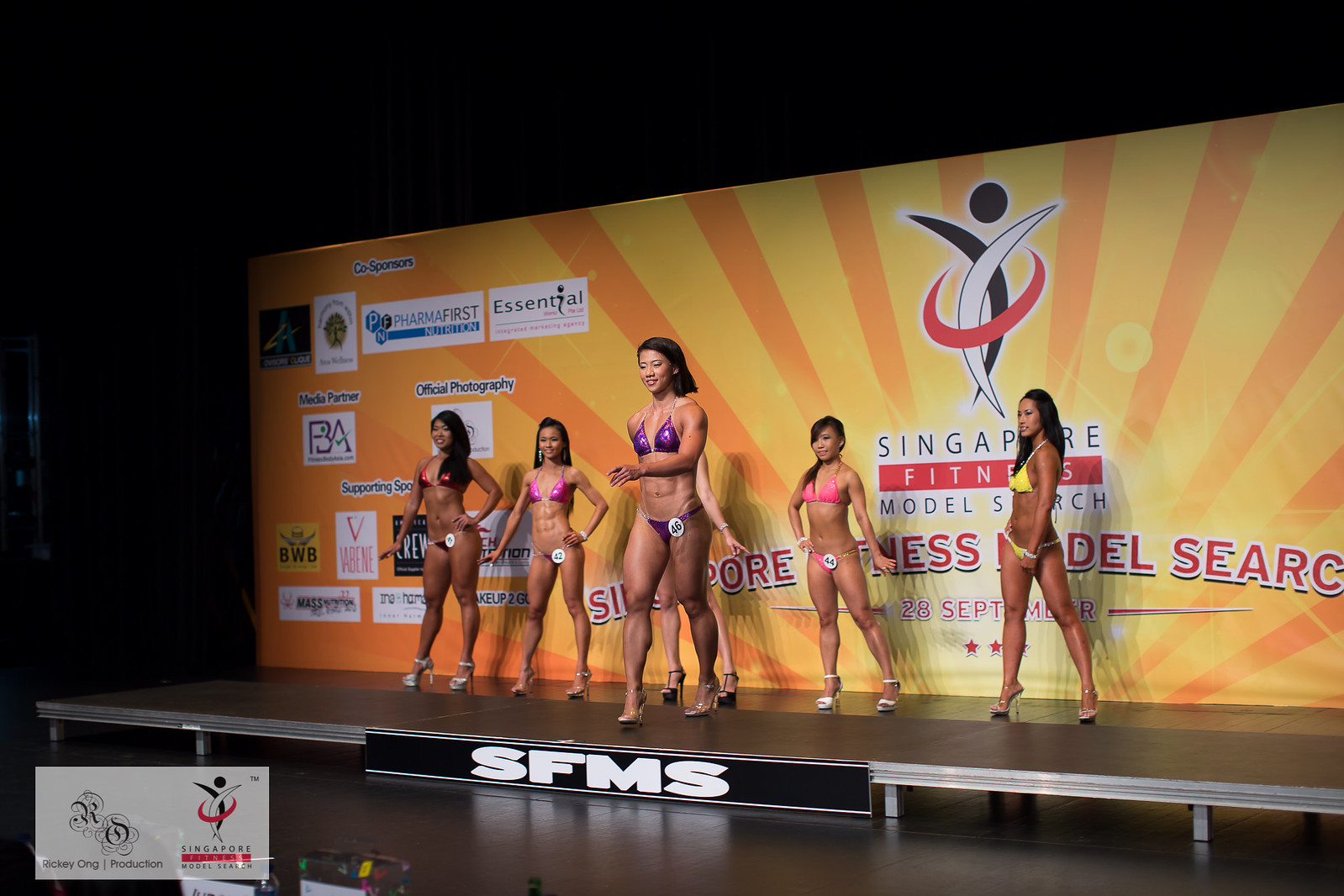The photograph captures six female fitness models, presumably of Asian descent, standing on an indoor stage during the "Singapore Fitness Model Search" event. They are all dressed in different colored bikinis and high heels, flaunting their well-toned bodies. The lady on the far left wears a metallic red bikini and white high heels. The second woman, who is slightly shorter, dons a shiny pink bikini with clear heels. At the center, a muscular female in a metallic purple bikini is walking forward; she has short black hair, wears black high heels, and bears the number 46. Behind her, partially visible, is another competitor. Moving to the right, there is another lady in a pink bikini with the number 44, followed by a seemingly teasing contestant in a yellow bikini, positioned sideways, with black hair and a bracelet. A black banner with silver edging adorns the front of the stage, emblazoned with the initials "S.F.M.S." in white letters. The stage wall at the back features vibrant orange and yellow sunburst stripes emanating from a central point, accompanied by multiple sponsor logos, including visible ones like "pharma first nutrition" and "Essential." The watermark on the bottom left corner of the image, though partially illegible, consists of a see-through white rectangle with two distinct logos. The judges' table is suggested but out of the frame, emphasizing the competitive nature of this fitness model search event.